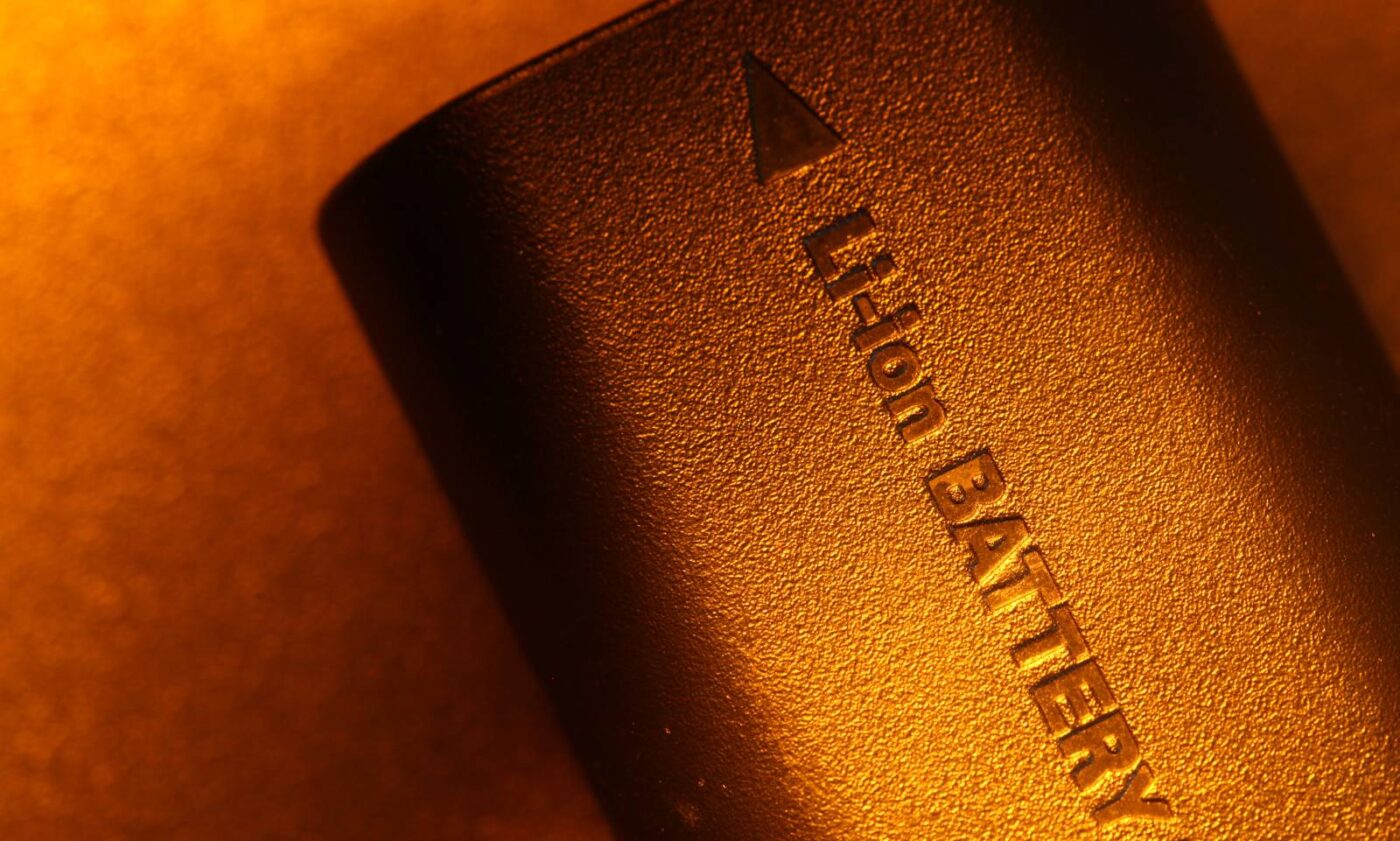The image features a prominent lithium-ion battery, clearly labeled with the text "LI-ION BATTERY," with each letter capitalized. The battery appears metallic and slightly rusted, positioned on a surface that is a mix of orange and brown hues. An arrow originates from the bottom right corner of the image, pointing diagonally towards the top center. The battery has a slightly curved shape with flat and illuminated surfaces, giving it a textured, highlighted appearance with hints of yellow light on the right side. The background is a blend of brownish gold and orange colors, adding depth to the scene.